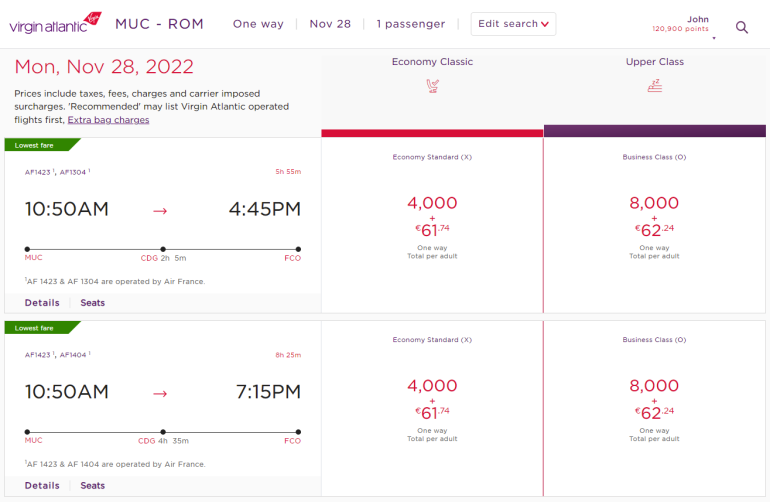The image is a screen capture of the Virgin Atlantic website, seemingly taken from a tablet, given the layout and display. The header showcases the Virgin Atlantic text in purple, while the tail logo, positioned to the right, features the word "Virgin" in pink. The flight details indicate a one-way trip from Munich (MUC) to Rome (FCO) on November 28th, with one passenger listed. There's an option to edit the search and a user named John is signed in, displaying a balance of 120,900 points. Additionally, a purple magnifying glass icon is visible, presumably for search functionality.

Below the header, highlighted in pink, the departure date, Monday, November 28th, 2022, is mentioned, with a note stating that prices include taxes, fees, charges, and carrier-imposed fees. The first flight option listed offers departure at 10:50 a.m. and arrival at 4:45 p.m. from Munich (MUC) to Rome (FCO). There are buttons for accessing more details and selecting seats. Another flight option shows departure at 7:50 a.m. and arrival at 7:15 p.m., noting differing durations.

Price options are categorized mainly under "Economy" and "Upper Class." The economy standard fare is listed at 4,000 points plus €61.74, while the business class fare (Upper Class) is 8,000 points plus €62.24. Both sets of options display identical prices for respective classes but differ in travel times. 

Though the information appears consistent, the details and layout give an impression of a mock-up due to the repetitive and evenly split fare structure across the economy and business classes. The referenced flight paths consistently show routes from Munich to Rome, adding to the unified but potentially mock-up appearance.